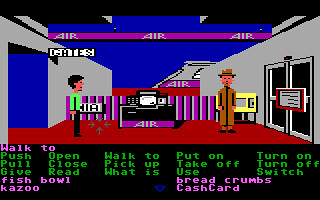This digital artwork features two characters positioned on either side of a central machine. On the left side, a person with black hair, dressed in a yellow shirt and black pants, is facing towards the center of the image. In the middle, there is a machine predominantly colored in black, with a white central section and gray accents below. To the right, another person is depicted wearing a brown hat. Text is present at the bottom of the image, adding context or narrative to the scene.